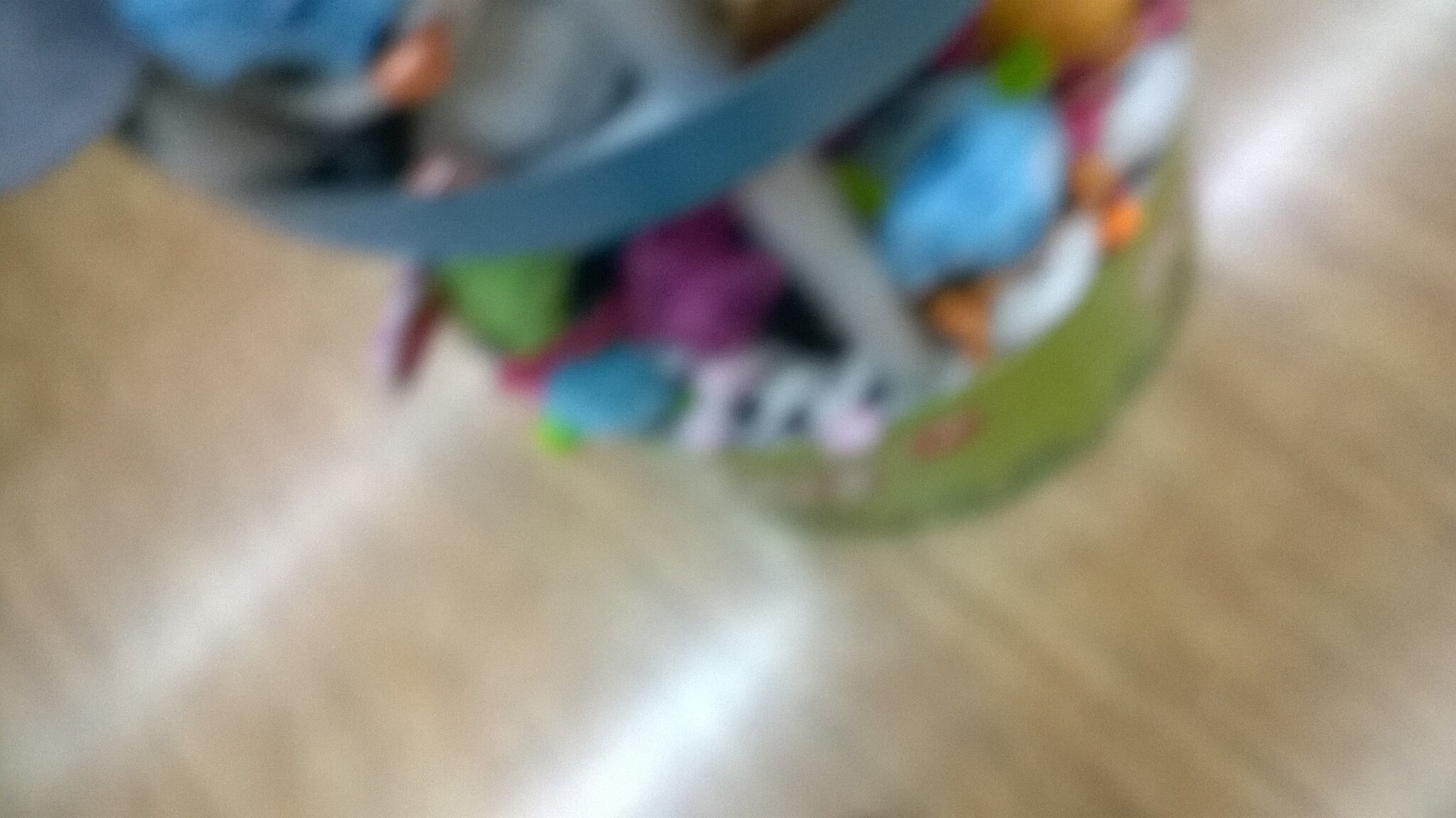This slightly blurry photograph captures a basket overflowing with children's plush toys. The basket sits on a highly polished, light wood-stained floor that gleams under the overhead lights. The toy basket itself features a distinctive design with a green band around its base, adorned with colorful images, possibly depicting flowers. Made from a loosely woven material, the basket allows for an easy view of the assorted plushies inside. Among the collection, a light blue plushie stands out, alongside a white plushie with black polka dots and a blue head. The open weave of the basket makes it simple to reach in and grab a toy, emphasizing its practical design. The ample light creates a sunny and cheerful atmosphere, highlighting the inviting nature of the play area.